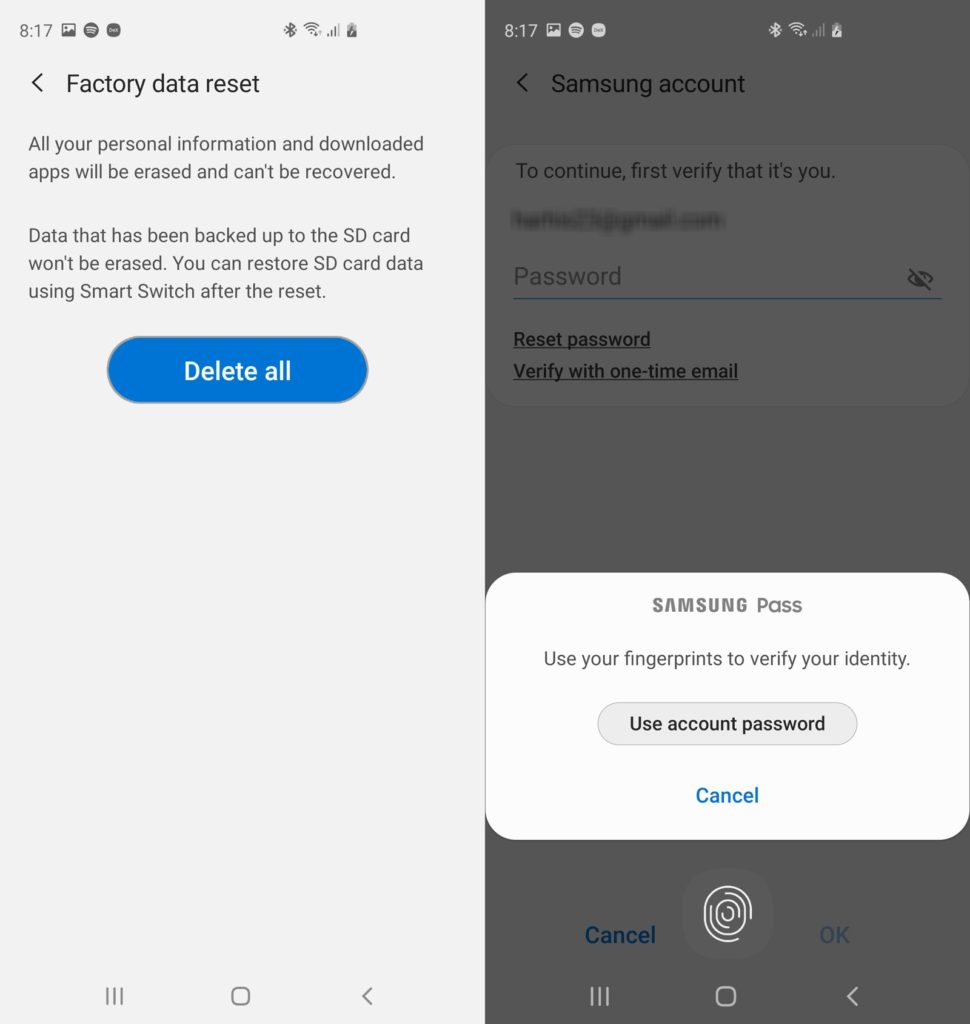**Caption:**

These side-by-side screenshots depict different stages of a smartphone reset and verification process. 

**Left Screenshot:**
- The background is light gray.
- The top bar displays icons for Bluetooth, Wi-Fi, cellular signal, and a battery indicator, all timestamped at 8:17.
- Below the top bar, a left arrow precedes the text "Factory Data Reset."
- A detailed paragraph explains that all personal information and downloaded apps will be erased and not recoverable, while data backed up to the SD card can be restored using Smart Switch after the reset.
- Beneath the paragraph, a prominent blue button labeled "Delete All" is visible.
- At the bottom of the screen, there are three navigation icons: three vertical bars, a circular square, and a left arrow.

**Right Screenshot:**
- The background is dark gray.
- Similar to the left, the top bar includes Bluetooth, Wi-Fi, cellular signal, and a battery indicator, also showing the time as 8:17.
- A pop-up menu with a white background appears near the bottom of the screen.
- The menu contains text starting with "Samsung Pass," followed by "Use your fingerprints to verify your identity," though some text is too small to read clearly.
  
The images offer a clear comparison between the factory reset instructions and the identity verification prompt using Samsung Pass.